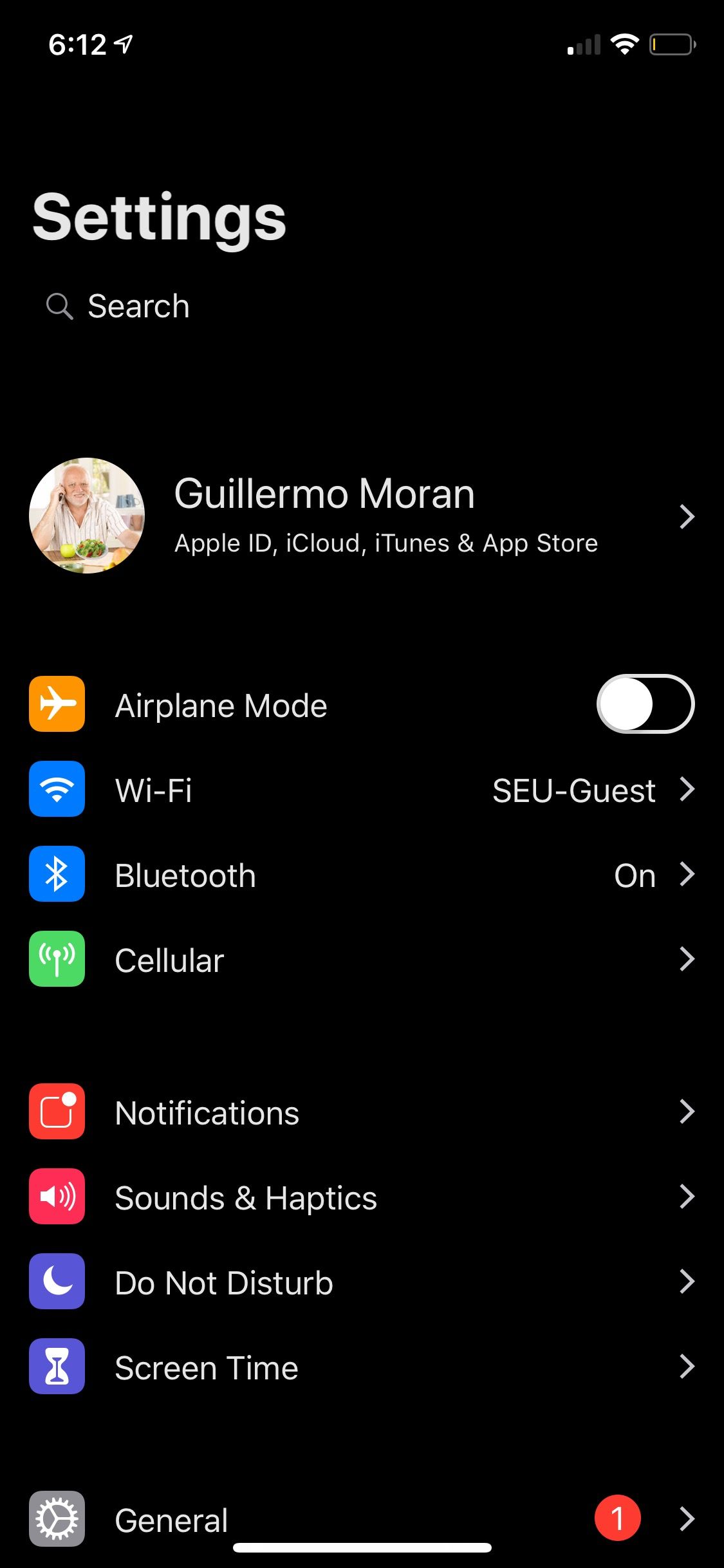A detailed screenshot from a mobile device, showing the time as 6:12, with one bar of cellular service and full Wi-Fi connectivity. The battery indicator shows a nearly depleted battery level, represented by a tiny sliver. The background is black with white text. At the top, it reads "Settings" followed by a search bar. Below the search bar, the text "Guillermo Moran" is displayed, accompanied by a profile picture on the left. Under "Guillermo Moran," it lists "Apple ID, iCloud, iTunes, and App Store," indicating the device owner's account information.

The settings menu begins with several selectable options:
- Airplane Mode: Currently switched off but can be toggled on.
- Wi-Fi: Connected to "SEU guest."
- Bluetooth: Turned on.
- Cellular: Option available for more settings.

Following these are further expandable options including:
- Notifications
- Sounds & Haptics
- Do Not Disturb
- Screen Time

At the very bottom of the settings menu is the "General" setting, with a red notification badge indicating one pending alert.